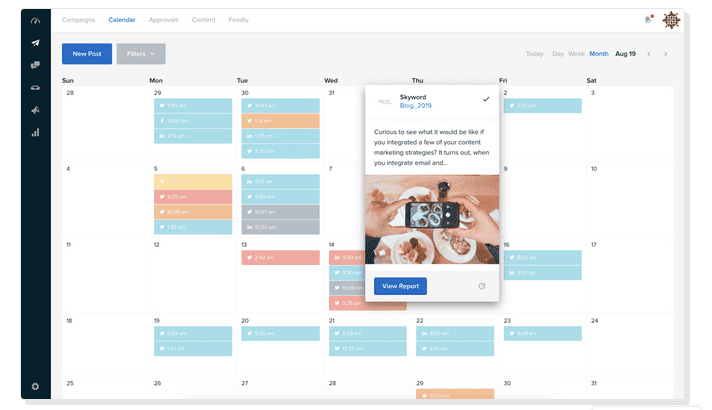The image consists of two overlapping screenshots on a white background. The screenshot on top is labeled "Skyward Blog" and features a query about integrating content marketing strategies, specifically mentioning email integration. Below this text, there is an image of an individual photographing their meal with a smartphone, accompanied by the phrase "View Report." 

The underlying screenshot appears to be a content calendar with several scheduled social media posts. Key details include:
- Monday the 29th: Posts scheduled for Twitter at 8:45 AM, Facebook at 10:00 AM, and Instagram at 2:15 PM.
- Tuesday: Another post for Twitter at 10:45 AM, with additional text in a foreign language and several sections marked with aqua-colored boxes.
- Friday the 2nd: A post scheduled for Twitter within an aqua-colored box.
- Monday the 6th: Posts scheduled for Twitter at 9:40 AM and Instagram at 10:27 AM, interspersed with various symbols of unclear meaning, possibly in a foreign language.

The overlapping top screenshot makes the underlying calendar difficult to read in full.